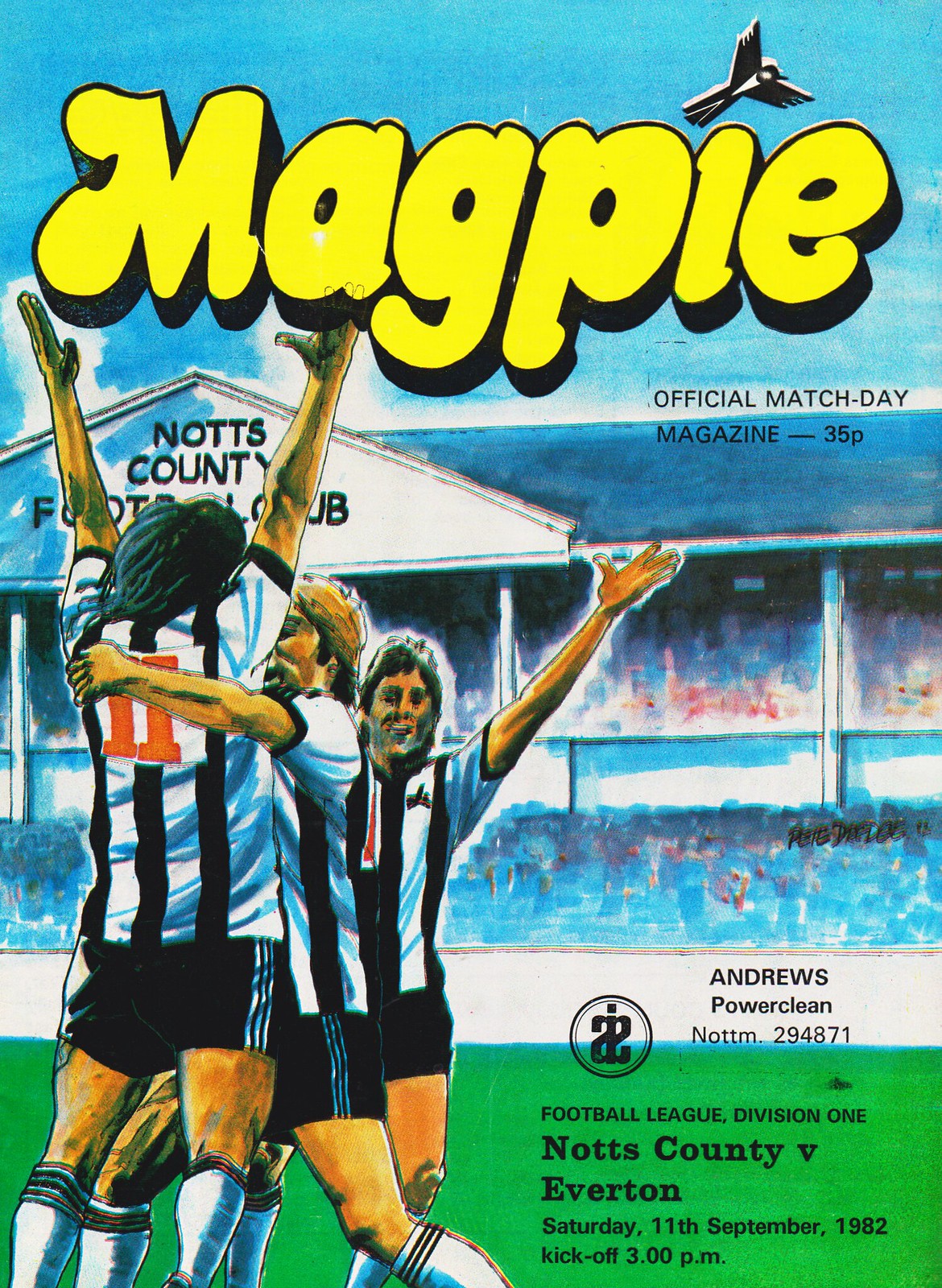The cover of this older, official Match Day magazine called Magpie is vividly illustrated and captures a celebratory moment of the Knott's County Football Club. Dominating the cover are three players in black and white striped jerseys with black shorts and white socks. One player is hugging another, while the third has his hands raised in the air, all set against a green soccer field. The background showcases a hand-drawn stadium with indistinct, muddled figures resembling cheering fans.

At the top, in large, yellow bubble letters, it spells "MAGPIE," with a small blackbird illustration perched above the letter "I." Just beneath, in smaller black text, it reads "Official Match Day Magazine 35P." Further down, text spans the cover indicating the event details: "Football League Division I, Knott's County v. Everton, Saturday, 11th September, 1982, kickoff, 3 p.m." Additionally, "Knott's County Football Club" is displayed on the roof of the illustrated stadium. Another prominent mention includes the sponsor, "Andrews Power Clean, Knottom, 294871." This rich, colorful artwork distinctly emphasizes the enthusiastic spirit of the football club and its supporters.